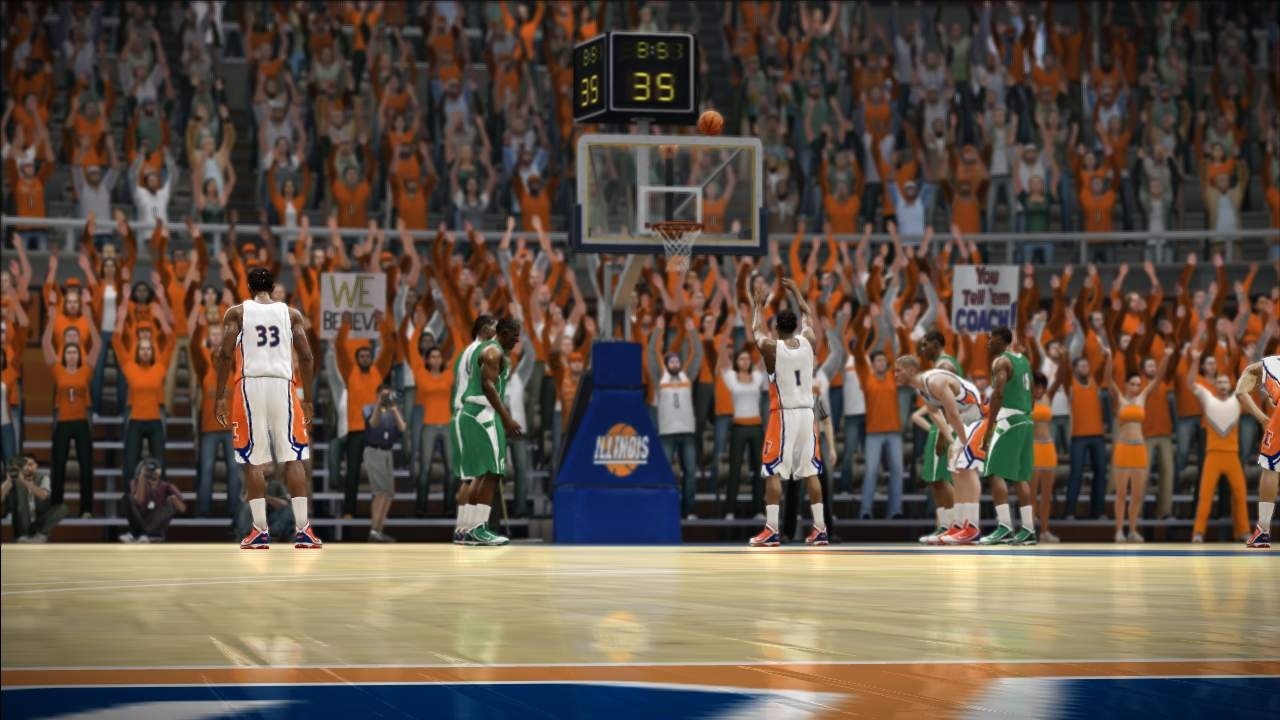This image captures a dynamic moment during a basketball game, evoking the surreal quality of a video game still. On the court, six players are visible, split evenly between two teams. The visiting team is outfitted in green shorts and matching jerseys, while the home team dons white jerseys with orange accents. The atmosphere is electric, with the stands awash in a sea of orange, clearly demonstrating the home crowd's enthusiastic support. At center stage, a player wearing jersey number 1 is poised at the free throw line, focusing intently as he releases the ball for a crucial free throw. Surrounding him, teammates and opponents alike are positioned strategically along the sides of the key, their eyes fixed on the ball’s trajectory. The tension in the scene is palpable, highlighting the significance of this moment in the game.